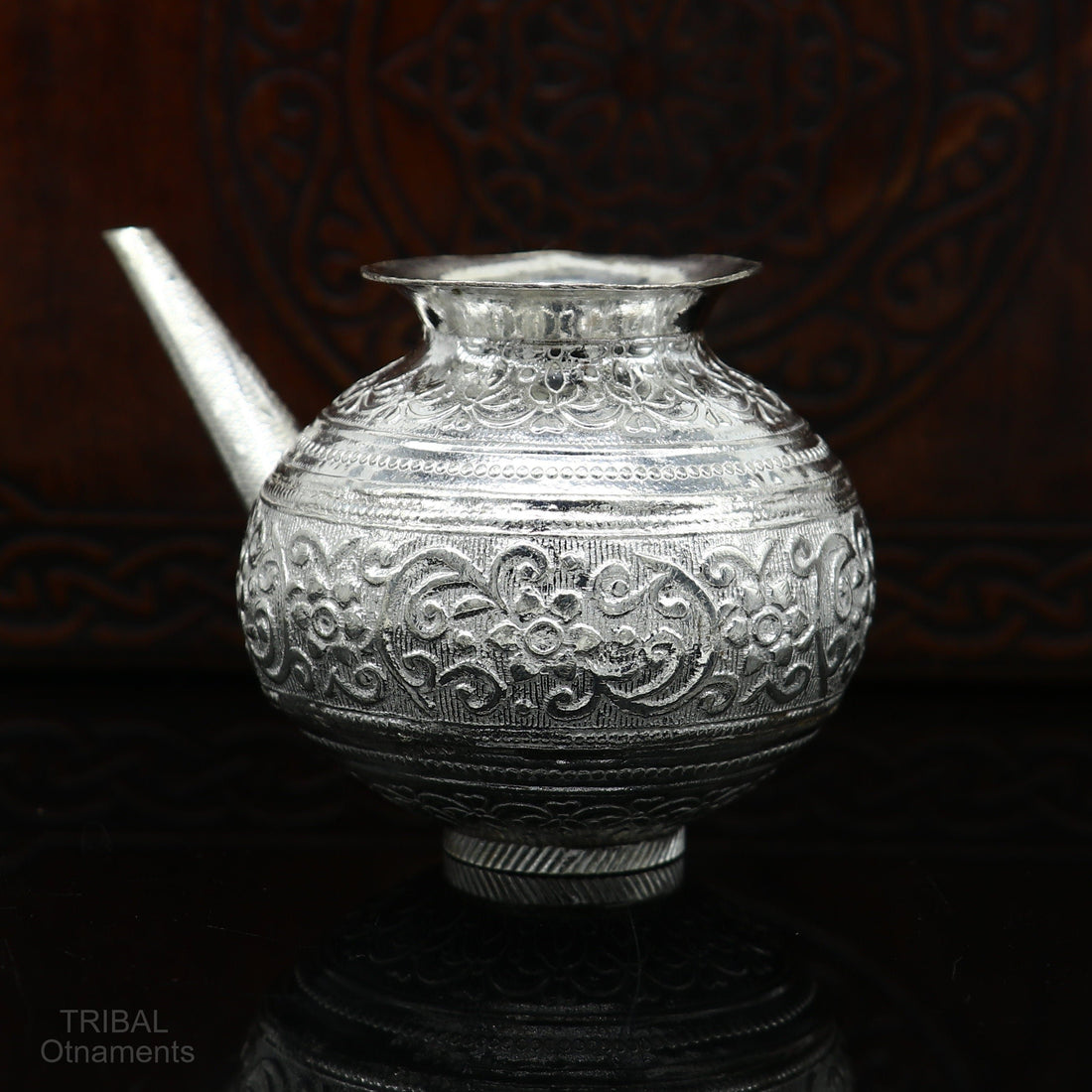A polished silver teapot, featuring a round and squat design, is prominently displayed in this photograph. The teapot has a deep body with a narrow base that expands to more than twice its width at its widest point before tapering back to form a graceful neck. On the side of the teapot, a curved spout extends, providing a functional and aesthetic element. The teapot rests on a dark, circular platform that appears to be another pot or a similar surface, adding contrast and depth to the composition.